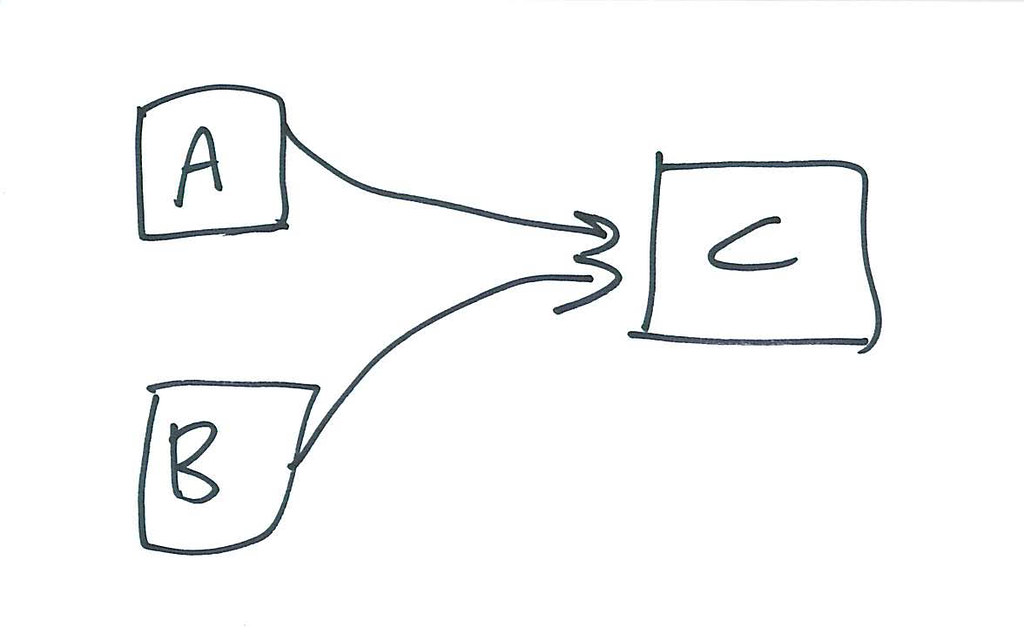This image features a hand-drawn diagram scanned into a digital format, set against a flat, computer-generated white background. The layout is simplistic but specific, showcasing three hand-drawn boxes and connecting arrows. 

- In the top left quadrant, there is a slightly uneven, hand-drawn box outlined in pen containing a capital "A."
- In the bottom left quadrant, another hand-drawn box appears—this time, more askew with a rounded bottom right corner—housing a capital "B."
- Slightly above and to the right of the "B" box, and positioned almost at the height of the "A" box, is a third hand-drawn box with a capital "C" inside.

Two arrows connect these boxes:
- One arrow originates from the right side of the "A" box, swoops downward and to the right, and points to the "C" box.
- Another arrow starts from the right side of the "B" box, curves upward and to the right, also directing towards the "C" box.

The lines and boxes show some waviness and imperfections, indicating that the diagram was quickly sketched by hand with minimal precision.